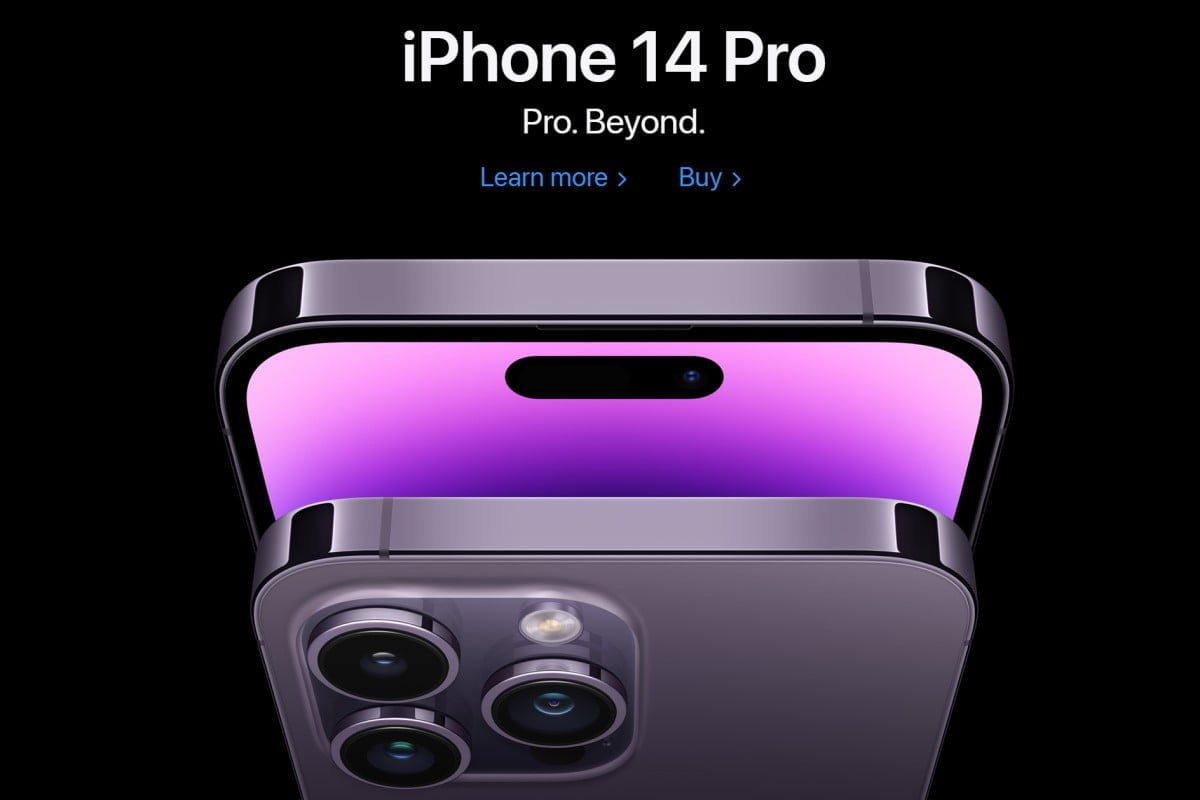The advertisement features the iPhone 14 Pro against a sleek black background. At the top of the image, white text reads "iPhone 14 Pro" followed by the tagline "Pro.Beyond." Beneath the tagline, there's a blue hyperlink labeled "Learn more" with a "Buy" option to its right. Centered below this text are two images of the iPhone 14 Pro. The first image showcases the front of the phone, highlighting a gradient purple screen that transitions from a light purple at the top to a dark purple at the bottom. Prominently visible are the front-facing camera and a black oval-shaped cutout, possibly housing the microphone. Encircling the screen is a sleek black border.

Adjacent to the front view, the second image displays the back of the phone, characterized by a grayish-purple hue. The back features three camera lenses and a flash, each accented by subtle glares that suggest either lighting effects or possible accent colors. The sides of the phone, however, do not reveal any buttons, leaving their presence uncertain.

Overall, the advertisement effectively emphasizes the premium design and advanced camera capabilities of the iPhone 14 Pro, capturing attention with its sophisticated color scheme and minimalist presentation.